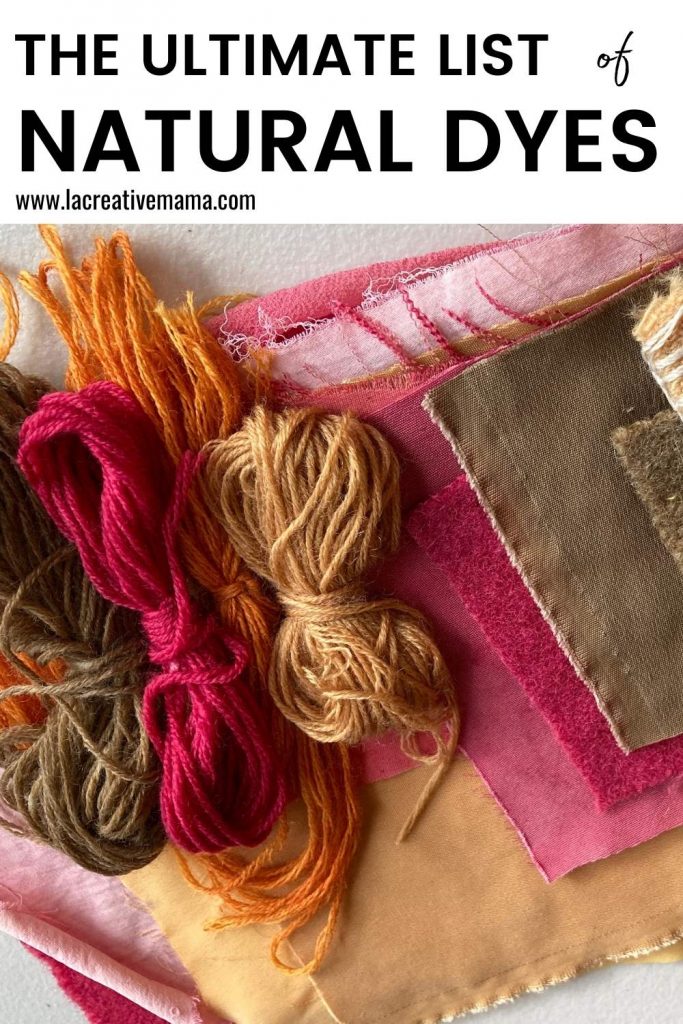The image is an advertisement for natural dyes featured on the homepage of www.lacreativemama.com. At the top of the image, the text "The Ultimate List of Natural Dyes" is displayed in black font on a white background, followed by the website address. Central to the image is a photorealistic display of four strands of yarn in different colors: brown, pink, orange, and light brown, all tied together in the center. These yarns are set against a layered backdrop of various fabric swatches in yellow, pink, purple, and light brown hues. The arrangement suggests a harmonious blend of materials and dyes, emphasizing the website's offerings in natural dyeing solutions.